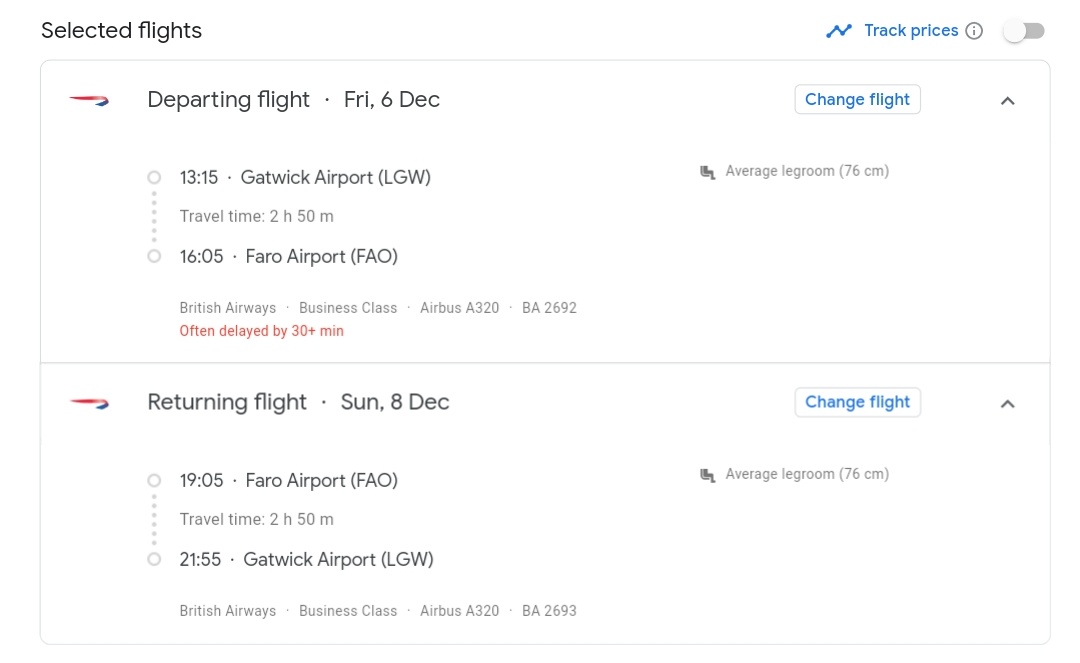The image depicts a detailed flight itinerary with various informational and interactive elements. In the upper left corner, it features the heading "Select Flights." On the upper right corner, a small line graph is shown alongside the blue text "Track Prices," with an information icon (a circle with an “i”) next to it. 

Adjacent to this text, there is a slider button for filtering flights, currently positioned to the left. The slider is represented by a white circle.

Below this section is the flight information. The first part details the departure flight, featuring a flight carrier logo on the upper left. It reads:

- **Departing Flight:** Friday, 6th December
- **Time:** 13:15, Gatwick Airport (LGW)
- **Travel Time:** 2 hours 50 minutes
- **Arrival Time:** 16:05, Faro Airport (FAO)
- **Airline and Class:** British Airways, Business class, Airbus A320 (Flight BA2692)
- **Status:** Often delayed by 30+ minutes (in red text)

In the upper right corner of this text box, there’s a "Change Flight" button in blue text. Additional information below this button mentions average legroom: 76 centimeters.

The second part details the return flight, including another carrier logo in red and blue. It reads:

- **Return Flight:** Sunday, 8th December
- **Time:** 19:05, Faro Airport (FAO)
- **Travel Time:** 2 hours 50 minutes
- **Arrival Time:** 21:55, Gatwick Airport (LGW)
- **Airline and Class:** British Airways, Business class, Airbus A320 (Flight BA2693)

Again, the upper right corner of the return flight text box has a "Change Flight" button in blue text and further mentions the average legroom: 76 centimeters.